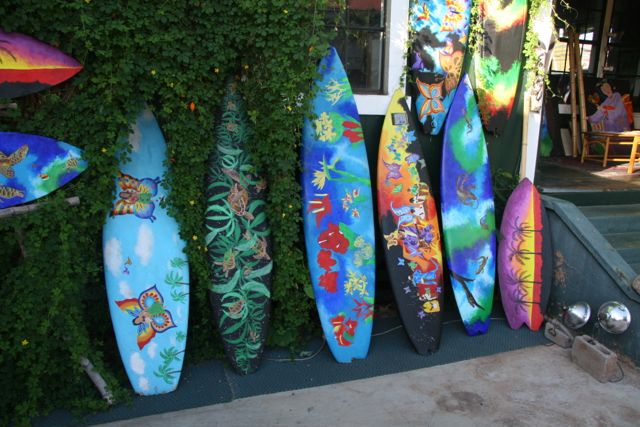This image depicts a vibrant, eclectic display outside what appears to be a beach-themed shop or café, characterized by its ornate surfboards. Leaning against a trellis adorned with ivy, eight surfboards boast stunning, hand-painted designs. The main arrangement features five full-sized surfboards and a smaller one leaning vertically, accompanied by the tips of two horizontally positioned boards in the upper left corner. Each surfboard showcases distinct artwork: 

- A surfboard with a pale blue background decorated with large butterflies and palm trees.
- Another with a dark green background, adorned with lighter green fronds and a vague, indiscernible animal.
- A vivid blue surfboard blooming with red, yellow, and green flowers.
- A black surfboard featuring an array of orange and yellow scenery interspersed with butterflies and other creatures.
- A mix of blue, white, green, and brown hues constituting another board.

Additionally, two surfboards hang vertically from the trellis, their vibrant colors partially visible. These include:

- One with the colors of magenta, yellow, and orange-red.
- Another striking one in vivid blue, aqua, and green tones.

A small, purple, yellow, orange, and black surfboard completes the collection, themed with a sunset and palm trees. Behind this picturesque display, a slightly blurry lady is seen sitting at a table near what appears to be the edge of a window. The scene hints at a welcoming atmosphere, possibly of a vibrant café or surf shop, complete with gray steps leading into the establishment. Overall, the display harmonizes the natural beauty of the surfboards with the quaint charm of the shop, inviting passersby into a colorful, beach-inspired haven.